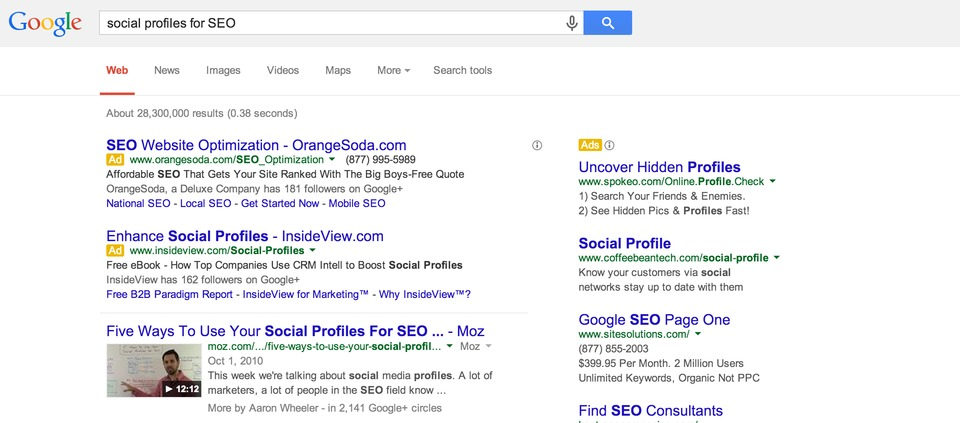Screenshot of a Google search result page for "social profiles for SEO." 

- **Header:** 
  - *Logo*: Google displayed in its characteristic alternating colors (blue, red, yellow, blue, green, red).

- **Search Query**: "social profiles for SEO."
  - **Tabs**: Web (selected), News, Images, Videos, Maps, More...
  - **Search Stats**: About 28,300,000 results (0.38 seconds).

- **Ad Results:**
  1. **Orange Soda SEO Website Optimization**
     - URL: orangesoda.com/SEO_optimization
     - Phone: 877-995-5989
     - Description: Affordable SEO that gets your site ranked highly. Free quote available. Orange Soda, a Deluxe company, has 181 followers on Google+. Services include National SEO, Local SEO, Mobile SEO.
  
  2. **InsideView Enhanced Social Profiles**
     - URL: insideview.com/social-profiles
     - Description: Free e-book on how top companies use CRM intel to boost social profiles. InsideView, which has 162 followers on Google+, also offers a Free B2B paradigm report and services aimed at marketing.

- **Organic Results:**
  1. **Moz Article: Five Ways to Use Your Social Profiles for SEO**
     - URL: moz.com/.../5-ways-to-use-your-social-profile
     - Date: October 1, 2010
     - Excerpt: Discussion on the importance and benefits of social media profiles in SEO. Written by Aaron Wheeler, who is in 2,141 Google+ circles.
     - *Note*: Includes a thumbnail from a 12-minute and 12-second video showing a man pointing at a whiteboard.

- **Additional Ads:**
  - **Spokeo**: Uncover hidden profiles at spokio.com.
    - Services: Search to find friends and enemies, view hidden pictures and profiles quickly.
  
  - **Coffee Bean Tech**: Social Profile services at coffeebeantech.com/social-profile.
    - Services: Connect with customers via social networks, stay updated.

  - **Site Solutions Google SEO Page**
    - URL: www.sitesolutions.com
    - Phone: 877-855-2003
    - Price: $399.95 per month
    - Description: Services include optimizing for organic searches, with 2 million users and unlimited keywords. No pay-per-click (PPC) included.
    - *Note*: Find SEO consultants link provided.

This detailed breakdown showcases the elements of the search results page, offering insights into available SEO services, helpful articles, and relevant advertisements.